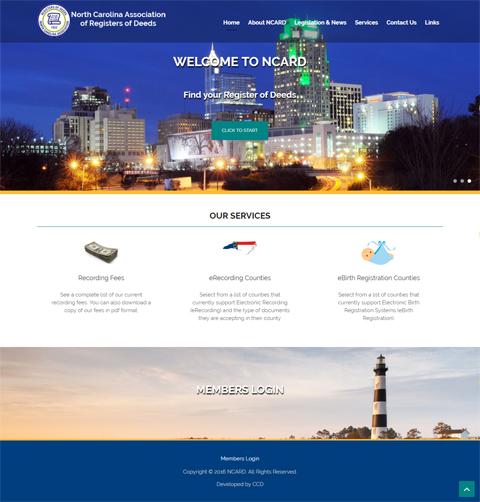The image depicts the official webpage of the North Carolina Association for Registration and Deeds (NCARD). Dominating the top of the webpage is a semi-transparent, blue navigation bar. This bar includes a small icon resembling a letter with a green circular outline.

The navigation menu, presented in white text, includes options: Home, About NCARD, Legislative Updates, News, Contact Us, and Links. Directly beneath the menu is a header image, presumably showcasing a cityscape from North Carolina, setting a welcoming tone with the text “Welcome to NCARD. Find your registration of deeds.”

A prominent green button with white text invites users to click and start their search for registration deeds. Below this header section, the main service offerings are listed against a white background with black text. These include:
- Recording Fees: Accompanied by an icon of a stack of money, with options to see the complete list of current recording fees and download them in PDF format.
- E-Recording Counties: Users can select from a list of counties that support electronic document recording.
- E-Birth Registration Counties: A list of counties that support electronic birth registration systems.

The page footer features an idyllic scene of a lighthouse with an adjoining small house surrounded by trees under a clear sky. Centrally placed in this serene image is a “Members Login” prompt, embellished with white lettering and a subtle black shadow background. 

At the very bottom of the page is a blue bar indicating “Members Login” and stating “Copyright 2016 NCARD. All Rights Reserved.” The footer also credits the site development to CCD and includes an upward green arrow button in the far bottom right corner.